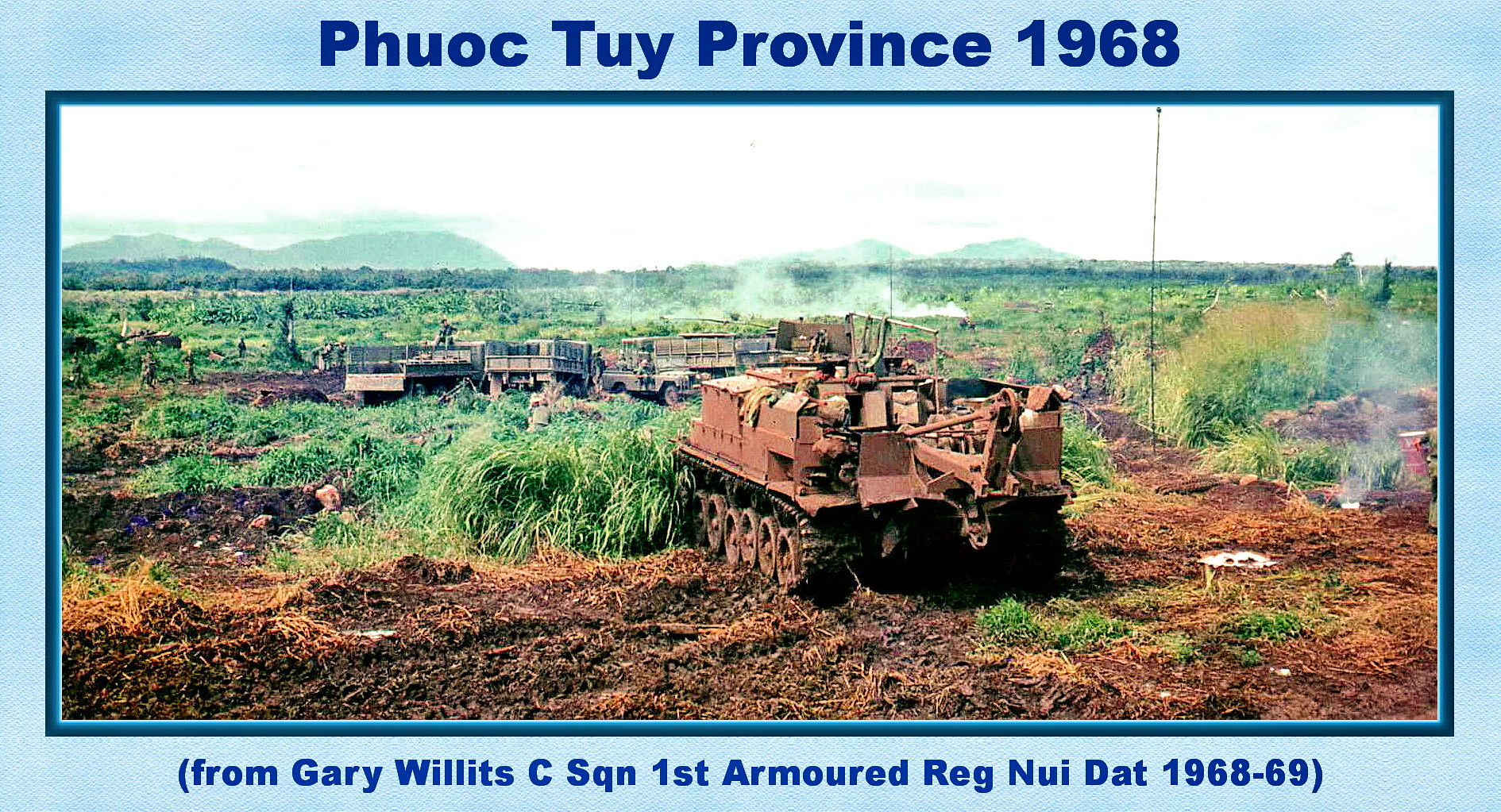This rectangular, vintage postcard-like photograph is framed with a light blue border and dark blue text. The top of the image reads "Phuoc Tuy Province, 1968," and the bottom caption states, "From Gary Willits, CSQN, First Armored Regiment, Nui Dat, 1968-69." The scene depicts a war-torn field that was possibly agricultural land, now dominated by military activity. Central to the image is a rusted or brown tank positioned on the edge of a mud pile, appearing to face the viewer. Surrounding the tank are several military vehicles, including a jeep in the background. The lower portion of the field features dark brown dirt, while the middle two-thirds are covered in varying heights of green grass. The horizon showcases a line of trees, extending to green, hilly terrain in the top left corner of the image. The sky above is hazy, suggesting a smoky or cloudy atmosphere, possibly indicative of recent fires or ongoing conflict. The entire composition evokes a vivid snapshot of the Vietnam War era, capturing both the natural and war-altered landscape of the time.